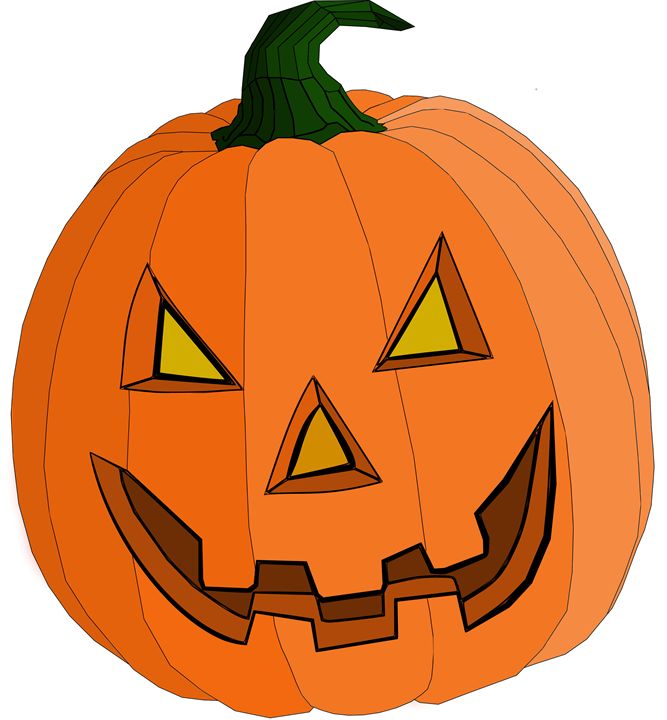This digital illustration depicts a jack-o'-lantern, meticulously rendered with very thin black lines for its outline and internal ridges, accentuating its form against a white background. The stem, characterized by slightly thicker sections in some areas, contributes a vibrant green hue that resembles a hat perched atop the pumpkin. The jack-o'-lantern sports an intimidating or mischievous expression, crafted through sharp, triangular eyes, a similarly shaped nose, and a jagged, pointed smile with three teeth on the top and two on the bottom. The eyes are illuminated with a dark yellow, while the nose features a duskier, browner shade of yellow; the mouth, however, reveals a dark interior. The pumpkin's orange surface displays various shades, with the front being more brightly colored than the lighter, subdued back. This illustration captures a blend of graphic precision and playful eeriness, typical of children's Halloween decorations.